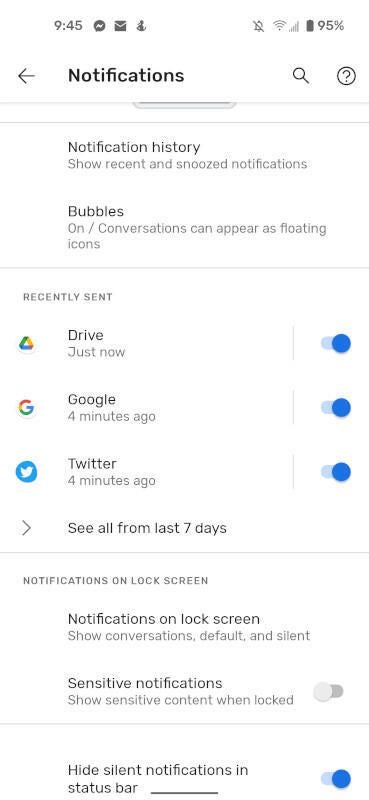In the image captured from a cell phone screen, the focus is on the "Notifications" settings menu. At the top of the screen, the word "Notifications" is prominently displayed with a left-pointing arrow, indicating the option to return to the previous menu. Below this, the "Notification history" section highlights the options to show recent and snoozed notifications. 

The next category is labeled "Bubbles," with a description indicating that conversations can appear as floating icons with the option turned "On." 

The "Recently sent" section follows, listing various apps and the timing of their notifications. "Drive" is listed with a notification from "just now," and the toggle switch beside it shows it is enabled. Google and Twitter both have notifications from "4 minutes ago," each with their respective toggles turned on. A link titled "See all from last 7 days" directs to a more comprehensive history and features a right-pointing arrow. 

Further down, the "Notifications on lock screen" section provides several settings. The first option, also named "Notifications on lock screen," is set to show conversations, defaults, and silent notifications. Below this, the "Sensitive notification" option, which controls the display of sensitive content when the phone is locked, is turned off. The last setting, "Hide silent notifications in status bar," is turned on, clearly indicated by a line separating these options from other settings.